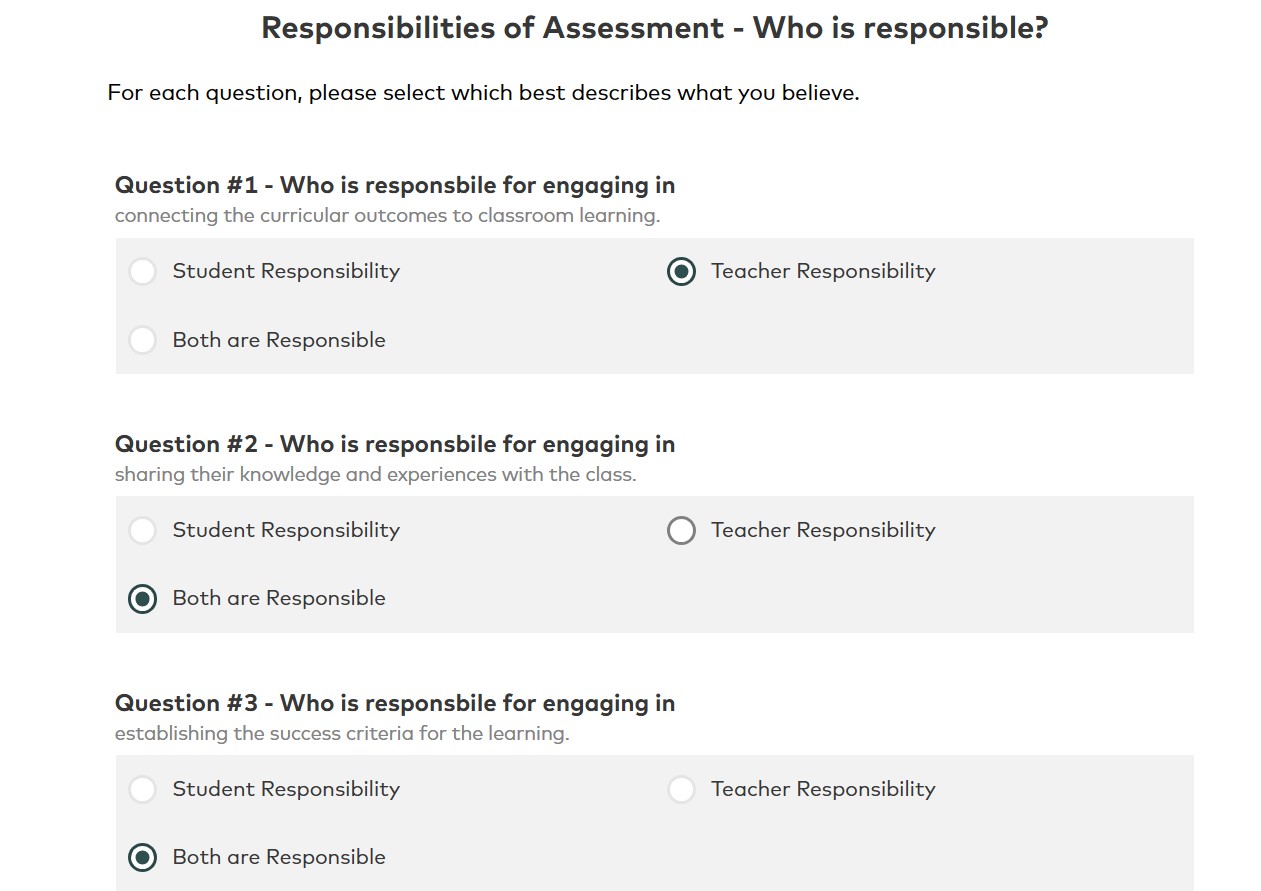A detailed and polished caption for the image could be:

"This screenshot showcases a questionnaire focused on delineating the responsibilities of assessment between students and teachers. At the top, the heading 'Responsibilities of Assessment' is displayed in black text, followed by an instruction: 'For each question, please select which best describes what you believe.' The questionnaire includes several questions, each accompanied by three response options: 'Student Responsibility,' 'Teacher Responsibility,' and 'Both Are Responsible.'

- **Question 1**: 'Who is responsible for engaging in connecting curricular outcomes to classroom learning?' The chosen response is 'Teacher Responsibility.'
- **Question 2**: 'Who is responsible for engaging in sharing their knowledge and experiences with the class?' The selected answer is 'Both Are Responsible.'
- **Question 3**: 'Who is responsible for engaging in establishing the success criteria for the learning?' Similarly, the response marked is 'Both Are Responsible.'

The respondents' selections indicate a belief in a shared responsibility for certain educational tasks, while assigning specific tasks primarily to teachers. Notably, the individual believes that both teachers and students should be involved in establishing success criteria for learning, although there is an opinion mentioned that this might ideally be a teacher's responsibility."